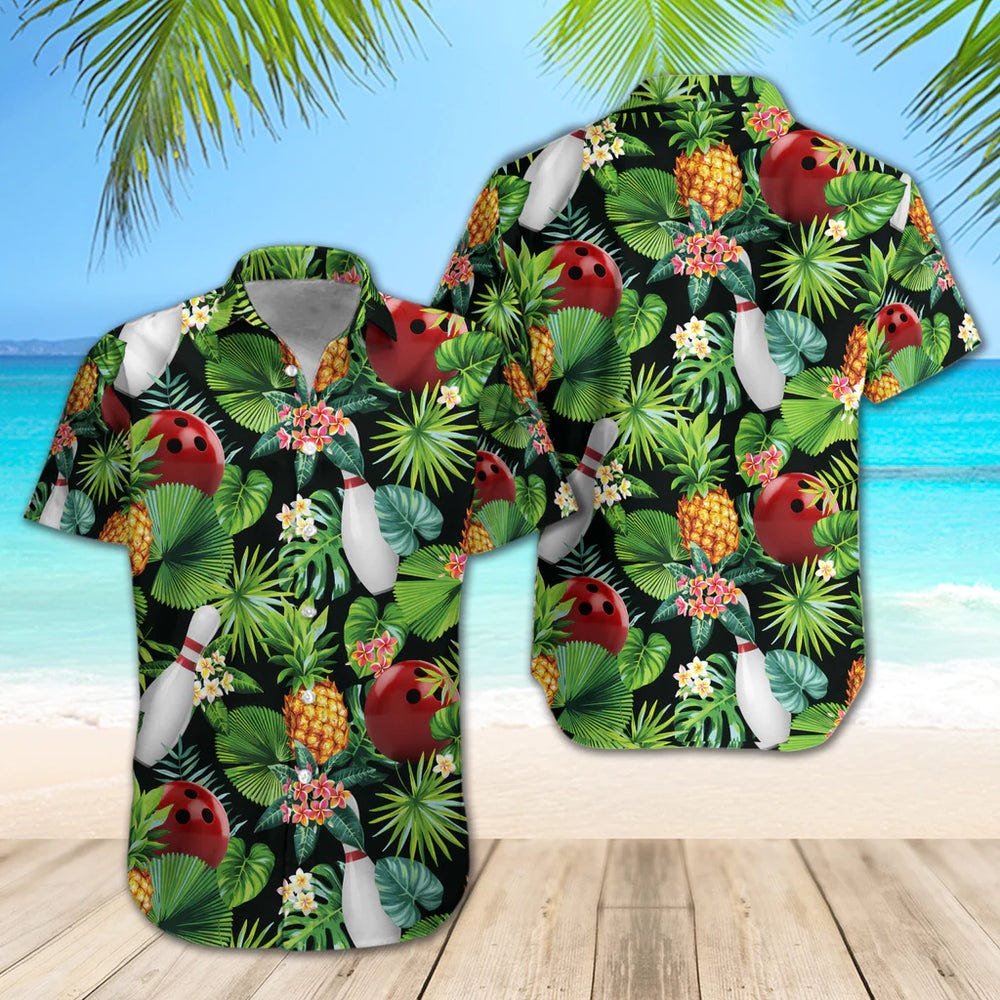This detailed image showcases the front and back of a vibrant, gaudy Hawaiian shirt set against a computer-generated tropical beach background. The left side features the front view, while the right side displays the back view of the same shirt, both suspended in midair. The background depicts a sunny, serene beach scene with the ocean meeting the horizon, pristine white sand, a small wooden boardwalk at the bottom, and palm tree leaves dangling from the top against a clear, blue sky.

The shirt itself is a bold explosion of green and is adorned with a distinctive tropical pattern, incorporating an array of leaves and fronds, along with playful elements such as bowling pins, bowling balls, and pineapples. The pins are white with two red stripes around their necks, the bowling balls are red with three holes, and the occasional tiny white and red floral buds are scattered throughout the design. Overall, the shirt embodies a dynamic and eccentric tropical, Hawaiian aesthetic.